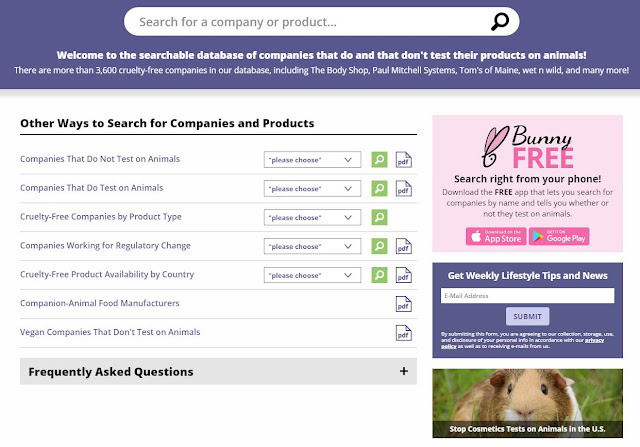The image depicts an interface with a muted blue strip running across the top, setting a calm yet professional tone. At the very top, there's a white search bar with gray text that prompts users to "search for company or product." To the right of the search bar is a black magnifying glass icon, inviting users to initiate their search.

Beneath the search bar, the interface features text in white font welcoming visitors to "the searchable database of companies that do and do not test their products on animals." It highlights that there are more than 3,600 cruelty-free companies in the database, including notable names such as The Body Shop, Paul and Michael Shell Systems, Palms of Maine, Wet and Wild, and many more.

Further down, the page presents additional options for searching companies and products. A section header in white font reads, "Other ways to search for companies and products," separated by a black line for clarity.

This section offers several dropdown menus, each aligned to the left:
1. "Companies that do not test on animals," accompanied by a green square and a magnifying glass icon, and a PDF link.
2. "Companies that do test on animals," with similar icons and dropdowns.
3. "Cruelty-free companies by product type," with a green square and PDF link.
4. "Companies working for regulatory change," also with a dropdown, green square, and PDF link.
5. "Cruelty-free product availability by country," featuring a dropdown, green square, and PDF link.
6. "Companion animal food manufacturers," with a PDF link.
7. "Vegan companies that don't test on animals," provided with a PDF link.

The organized layout, clear headings, and helpful icons ensure that users can easily navigate and access the information they need.